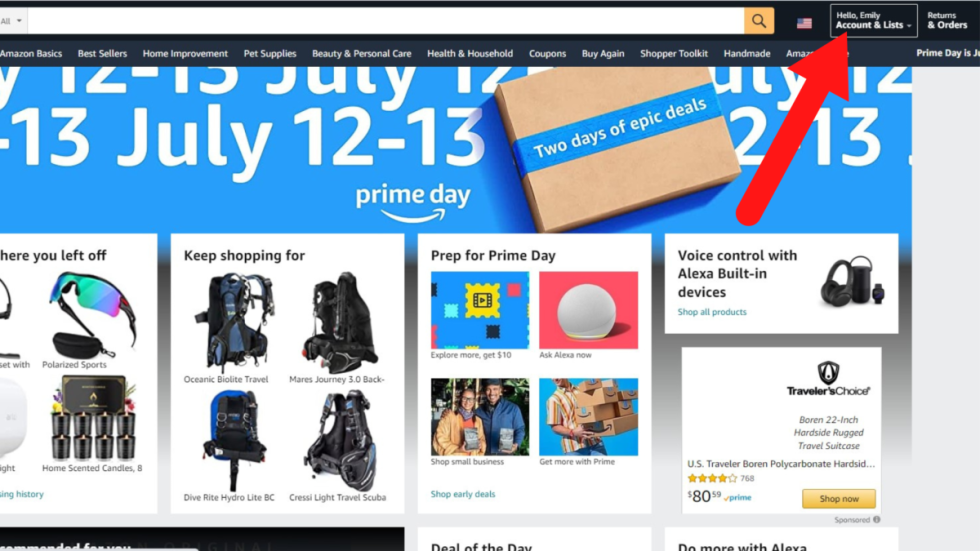This image is a screenshot of the Amazon.com homepage. At the very top is a prominently displayed search bar, which features a yellow magnifying glass icon in the right-hand corner. To the right of the search bar, there is an American flag followed by a box greeting the user with "Hello, Emily." This box includes a drop-down menu for account options and links. A red arrow is superimposed on the screen, pointing directly to the "Hello, Emily" box. Adjacent to this box is a hyperlink for returns and orders.

Below this header section, a series of navigation links starts from the left-hand side: 
- Amazon Basics
- Best Sellers
- Home Improvement
- Pet Supplies
- Beauty and Personal Care
- Health and Household
- Coupons
- Buy Again
- Shopper Toolkit
- Handmade

The next link in the sequence is obscured by the red arrow, making it unreadable. 

On the far right of the header, there is a partial sentence promoting Prime Day: "Prime Day is June," which is incomplete as the end date is cut off. Below this header, a blue banner announces the Prime Day dates, "July 12-13th," accompanied by an image of a box with packing tape that reads, “Two Days of Epic Deals.”

The content below the banner features a section titled "Where You Left Off," displaying a pair of polarized sunglasses under "Polarized Sports" and an 8-pack of black candles under "Home Synthetic Candles." Adjacent to this section is another segment titled "Keep Shopping For," which shows various backpacks:
- Oceanic Bio-Lite Travel Backpack
- Mary's Journey 3.0 Backpack
- Diverite Hydro-Lite BC
- Cressi Lite Travel Scuba Backpack

Following these sections, there are two highlighted boxes:
- One labeled "Prep for Prime Day."
- Another titled "Voice Control with Alexa Built-in Devices."

On the far right, an ad for "Traveler's Choice Borin 22-inch hard-side rugged travel suitcase" indicates a sale price of $80.59 with Prime, alongside a yellow "Shop Now" button. Notably, the image for this ad is missing.